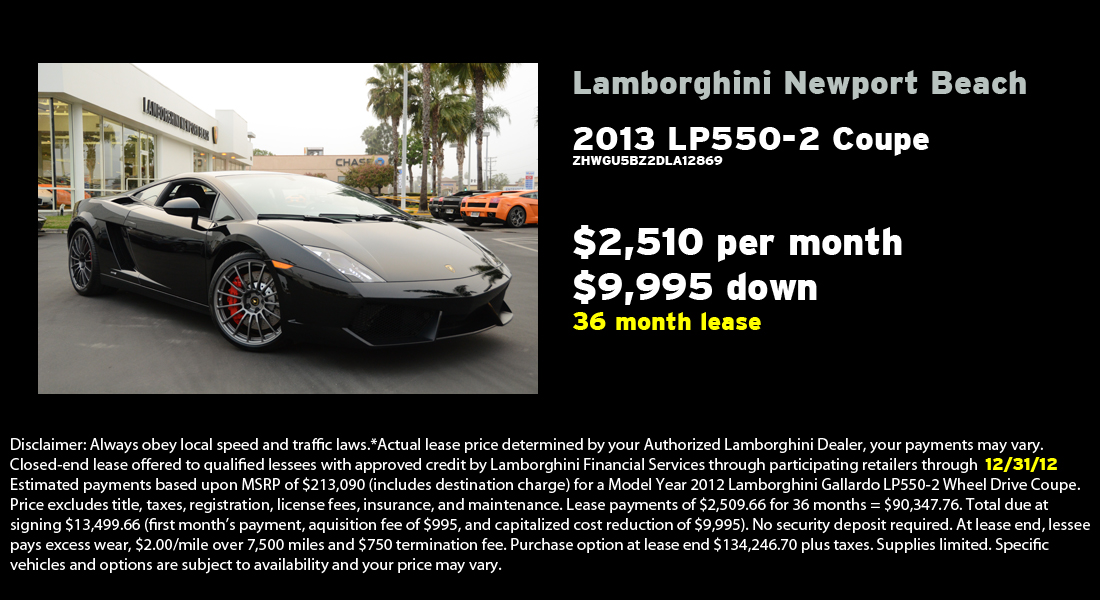The advertisement features a black Lamborghini LP 550-2 parked outside a Lamborghini dealership, likely Lamborghini Newport Beach. In the background, there are palm trees and additional Lamborghinis, indicating a luxurious and exotic location. The ad is dominated by a rectangular black graphic, making the image wider than it is tall. 

On the left side of the graphic is the photograph of the Lamborghini, with the dealership's name and logo visible at the top of the building. The right side displays details of the lease offer: "Lamborghini Newport Beach 2013 LP 550-2 Coupe, $2,510 per month with $9,995 down for a 36-month lease." Below this, a vehicle identification number (VIN) is partially mentioned: "ZHWGU5BZ2DLA12869." The bottom quarter of the advertisement contains a white text disclaimer, emphasizing the need to obey traffic laws and noting that actual lease terms and vehicle availability may vary based on dealership and options chosen.